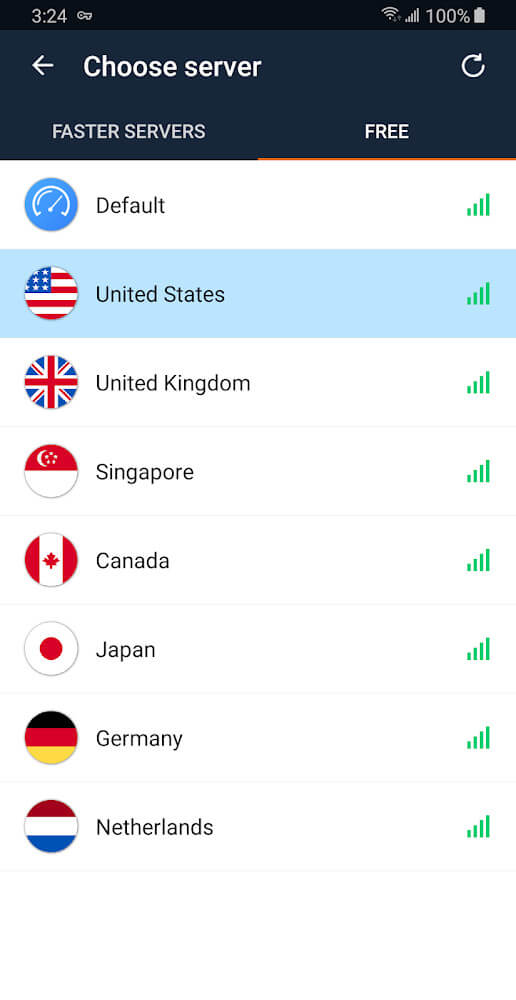The image depicts the screen of a person's cell phone, displaying a VPN application interface. The time at the top of the screen is 3:24, and the battery indicator shows a full charge at 100%. At the top-left corner, there is a back arrow labeled "Choose Server," implying navigation to server selection. Below this, the text "Faster Servers" appears, accompanied by the word "Free" on the right side.

The server selection area features eight circular icons, each representing different countries. To the right of each country's icon, four green bars indicate the connection strength. 

1. The default selection is the United States, highlighted with a blue circle and showing the US flag. 
2. Next listed is the United Kingdom with its flag displayed.
3. Following that is Singapore, represented by a white and red circle.
4. Canada is shown with its distinctive maple leaf flag.
5. Japan's icon includes a white background with a red dot.
6. Germany's icon features black, red, and yellow colors.
7. The Netherlands is indicated with red, white, and blue stripes.

All icons appear in a vertical list, facilitating easy selection for the user.